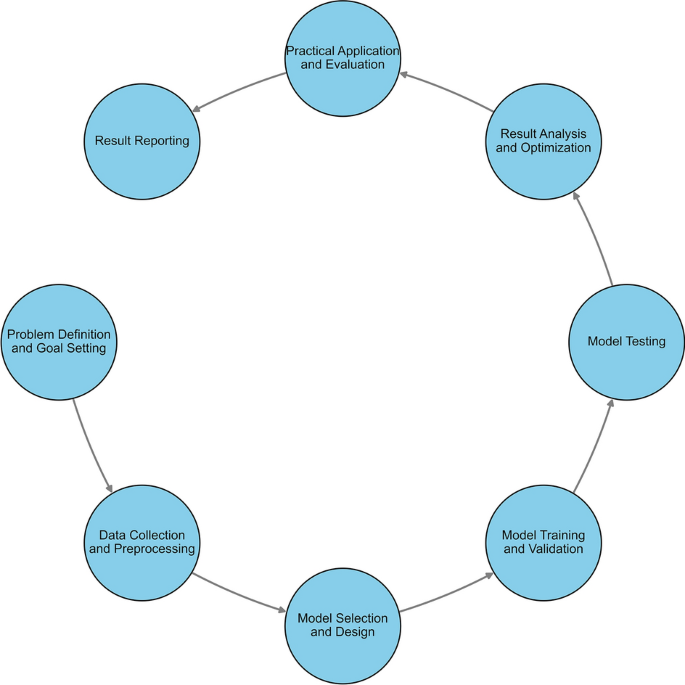The image displays a simple, circular flow chart composed of blue circles with black borders and black text. The chart outlines a sequence of steps often seen in a scientific or procedural context, depicted with each circle connected by an arrow pointing to the next. Starting from the left, the steps are as follows: "problem definition and goal-setting," leading to "data collection and pre-processing," followed by "model selection and design," progressing to "model training and validation," then "model testing," moving to "result analysis and optimization," followed by "physical application and evaluation," and concluding with "results reporting." All elements are arranged in a counterclockwise direction, and the center of this circular arrangement is white, giving a clean and uncluttered look to the chart.